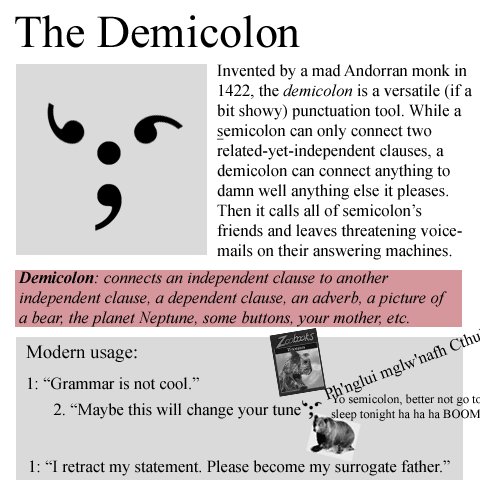This image is a screenshot from a digital book page explaining the "demicolon." The demicolon, illustrated here as three commas arranged in a triangular formation around a central period, was invented by a mad Andorran monk in 1422. Described as a versatile and flamboyant punctuation mark, the demicolon is noted for its flexibility, allowing it to connect any elements it chooses, unlike the semicolon, which can only connect two related but independent clauses. The passage humorously mentions that the demicolon even leaves threatening voicemails to the semicolon's friends. Highlighted in pink, additional information states that the demicolon can link an independent clause to another independent clause, a dependent clause, an adverb, a picture of a bear, the planet Neptune, some buttons, your mother, etc. The page also features a section on modern usage with examples accompanied by a picture of a bear.